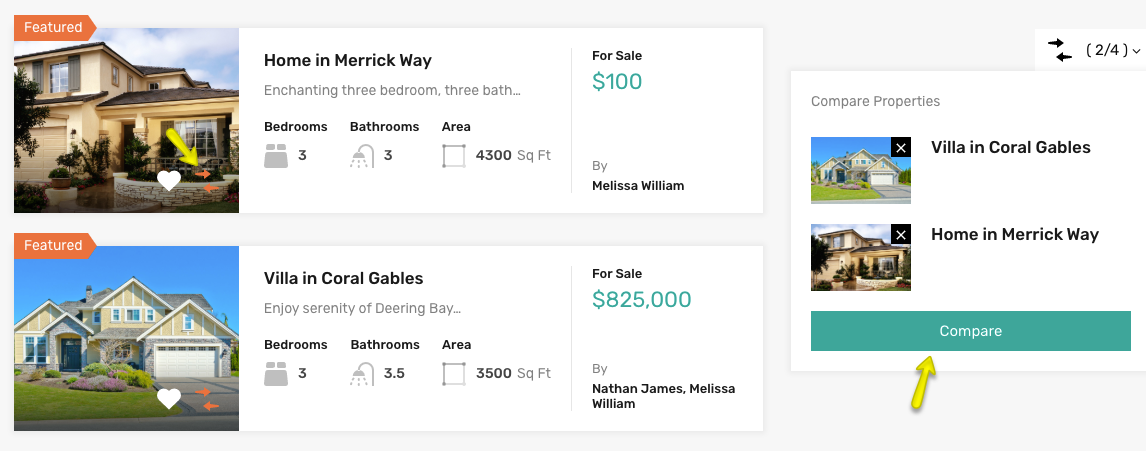Screenshot of a Realty Website Featuring Two Homes

The screenshot captures a section of a realty website, identified by its clean design and emphasis on property listings. 

In the upper left corner, a property image showcases a modern, tan house with a black roof. An orange label marked "Featured" overlays this picture. To the right, the text reads: "Home in Merrick Way For Sale" followed by "100 dollars," though this is likely an incomplete price listing. The detailed specifications of this home are provided: three bedrooms, three bathrooms, and areas measuring 2,400 and 4,300 square feet respectively. Further details reveal the listing agent, "By Melissa William."

Below this, another white rectangular section displays a second featured property. This image highlights a substantial yellow house with an attached garage. It is similarly distinguished with the orange "Featured" label in the upper left corner. The listing states: "Villa in Coral Gables, Enjoy Serenity of Deering Bay, For Sale $825,000." This villa offers three bedrooms, three and a half bathrooms, and an area of 3,500 square feet. The listing agents for this property are noted as "Nathan James and Melissa William."

On the right side of the screenshot, a smaller square labeled "Compare Properties" presents images of both homes, though their positions are swapped compared to above. The label reads "Villa in Coral Gables" for the top house and "Home in Merrick Way" for the bottom house. A prominent green rectangle below this section features the text "Compare," accompanied by a yellow arrow pointing towards it, suggesting an interactive feature for comparing the two properties.

Overall, the screenshot provides a detailed glimpse into a realty website, highlighting the features and agents for two attractive homes.